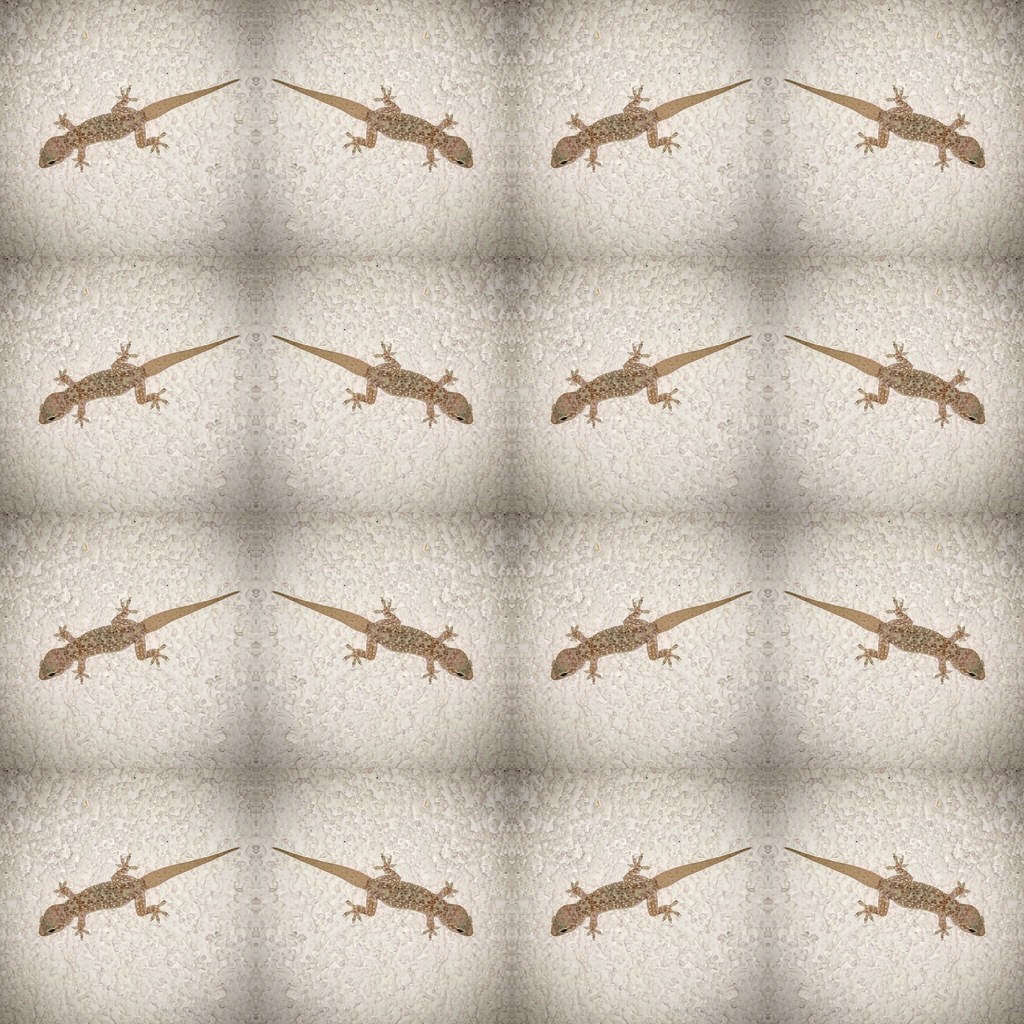This detailed image features a series of 16 identical depictions of a small tan, greenish-brown lizard, likely a gecko or salamander. Each individual lizard is meticulously drawn or painted with intricate detail, highlighting the textured bumps on their bodies and their small toes. The lizards are placed within a 4x4 grid of squares. Each square alternates the lizard's position; heads and tails are flipped in a repetitive pattern, creating a dynamic visual effect. The background of each square is a stone-textured beige cream color, adding a subtle, unadorned backdrop that emphasizes the lizards' details. The overall composition is very simple and plain, yet rich in texture and pattern, suggesting that the artwork might have been crafted on a stone-like surface.